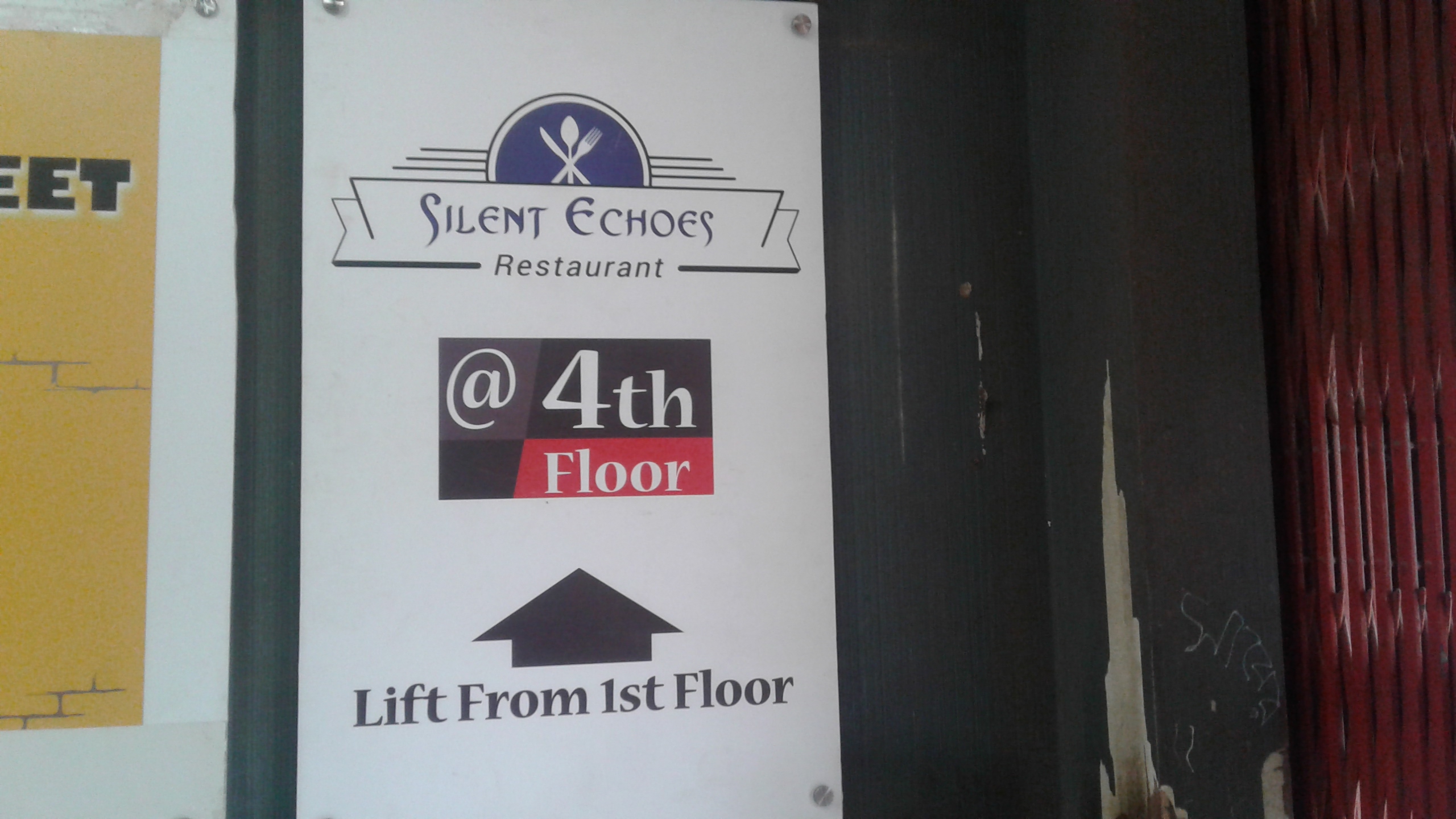The photograph captures an exterior scene featuring a prominent sign for the Silent Echoes Restaurant, a multi-story establishment advertised to be located on the fourth floor. The sign, set against a white background, displays a purplish text that reads: "Silent Echoes Restaurant" accompanied by a distinct logo of a knife, spoon, and fork crossing each other. Below this logo, the text "At Fourth Floor" is presented on a black horizontal rectangle, with the word "Floor" highlighted in red and "Fourth" in white. Beneath this lies an upward-pointing arrow with the instruction, "Lift from First Floor" written in black. The sign is partially set against a brown wooden building structure to the right, and a cut-off yellow sign to the left reading "EET." Surrounding the sign, the building seems worn with chipped paint and sporadic graffiti, particularly noticeable near a 90-degree corner composed of two black sections marred with gray patches. Adding to the atmosphere, red vertical stripes accent the right-hand side of the wall, emphasizing the run-down and weathered condition of the setting. The overall colors in the scene include yellow, white, black, gray, blue, off-red, maroon, and brown, contributing to a somewhat chaotic yet engaging visual experience that suggests an older, possibly neglected urban area.